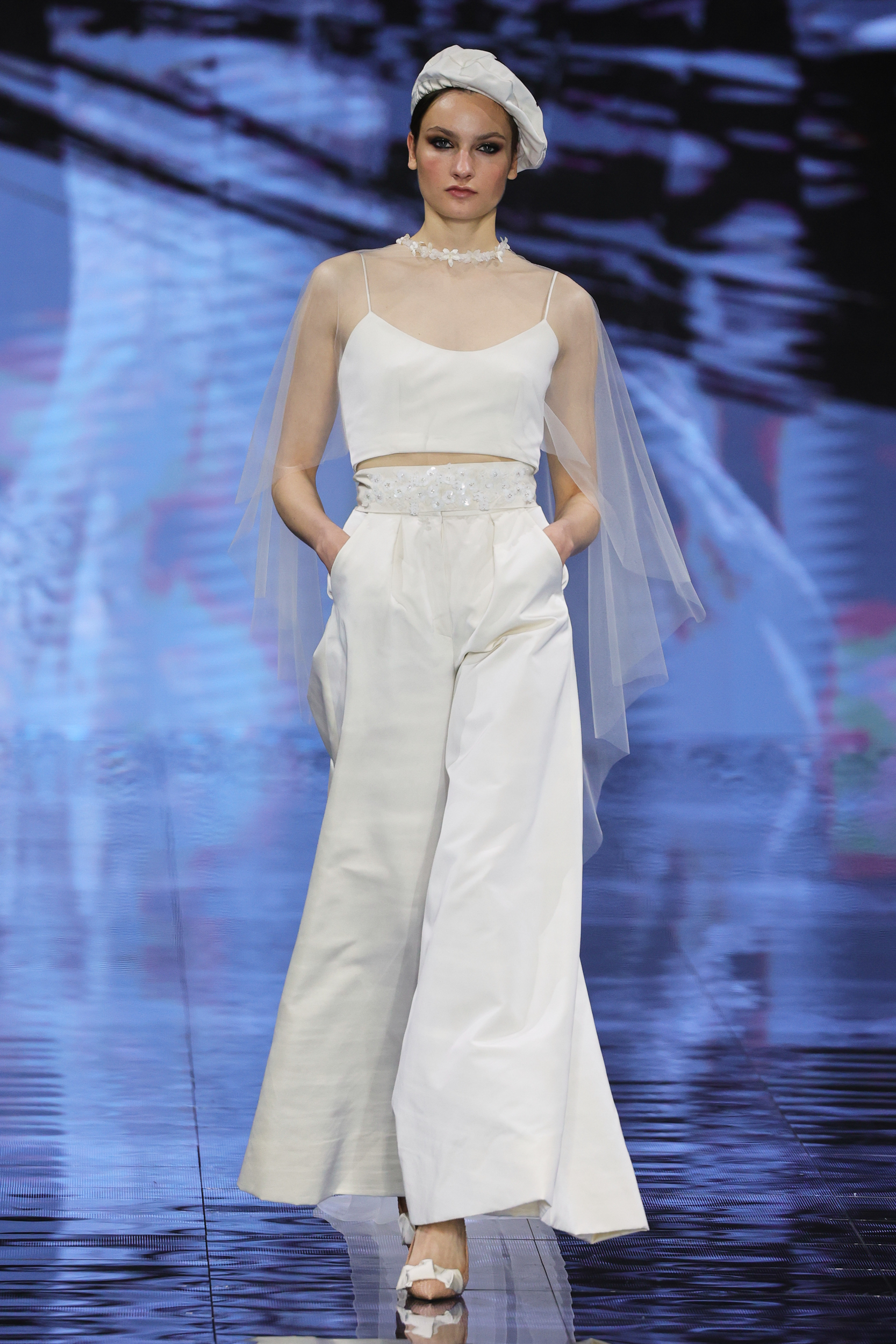This high-quality photograph captures a model, a fair-skinned brunette, confidently striding forward on a sleek, possibly touchscreen-like runway, tiled in large, smooth tiles with subtle ripples under her feet. She is entirely clad in white, exuding elegance in a decorative white cap that resembles a French beret and a striking necklace, possibly made of rhinestones or flowers, which adds to her sophisticated appearance. Her outfit consists of a white spaghetti-strapped crop top, over which she drapes a delicate, sheer cape that cascades down to her waist. This cape is adorned with intricate embellishments around the neck. She sports a wide, rhinestones-embellished belt that cinches her high-waisted, flourishy, satin trousers, which are so wide-legged they almost appear to be a skirt. Her trousers have deep pockets where she casually rests her hands. Completing her look are pointed-heeled shoes, adorned with a charming white bow on the toe. She's poised with heavy eye makeup, featuring lots of mascara, very arched eyebrows, and a moderate amount of lipstick and blush, delivering an overall fierce and stylish presence. The background is slightly blurred, ensuring all attention remains on her chic ensemble and confident demeanor.